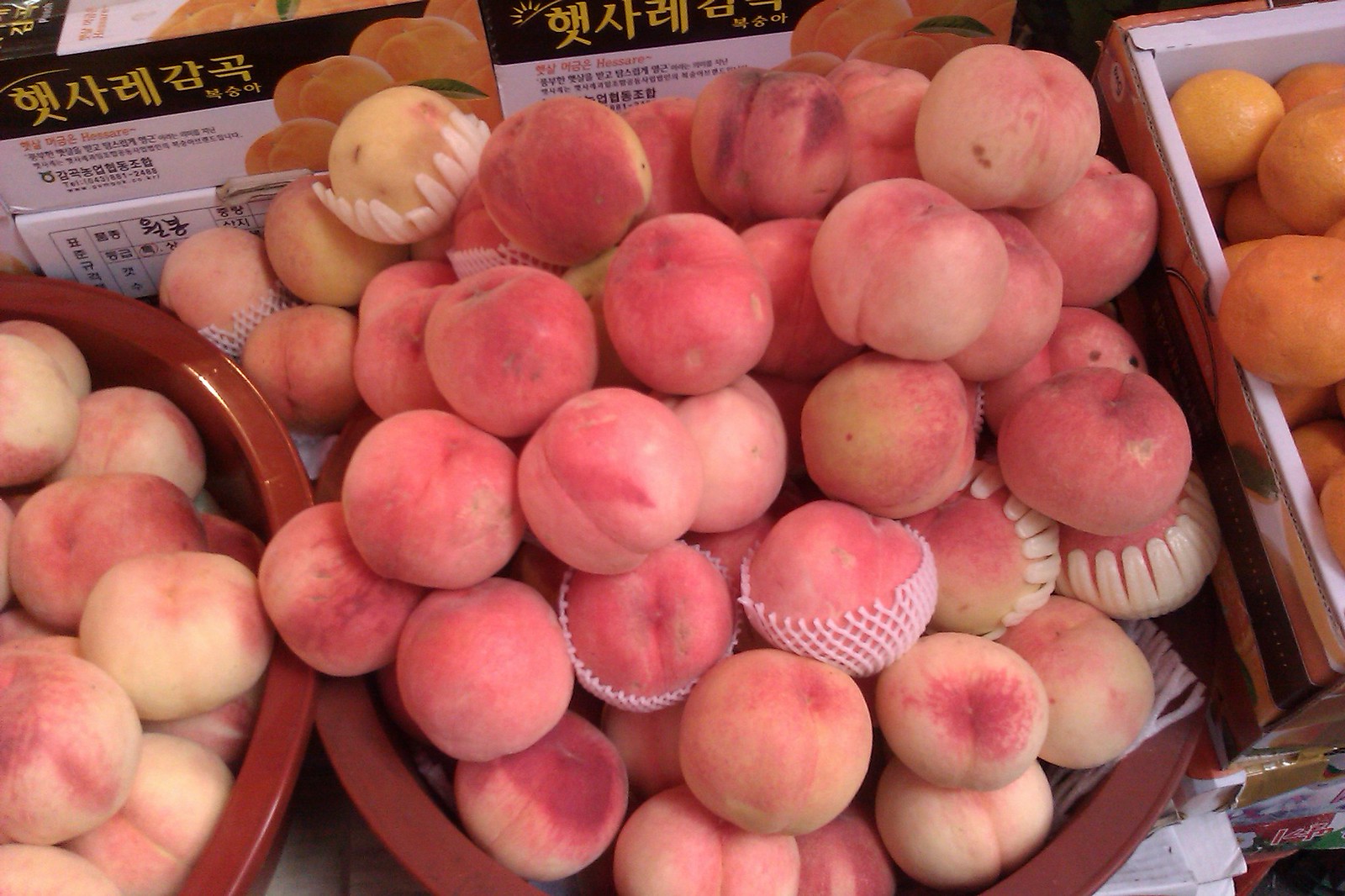This color photograph, likely taken at a supermarket or farmer's market, showcases a vibrant display of peaches and other fruits. Dominating the image are two large bowls filled with ripe peaches, displaying shades of pink, red, and tepid tan. Some peaches are encased in protective white netting or plastic picket-like wraps. To the right, partially out of the shot, there's a white cardboard box containing either oranges or nectarines. In the background, several boxes and crates with Chinese lettering are visible, suggesting the original packaging for these fruits. The vividly detailed scene captures the abundance and variety of the produce on display.